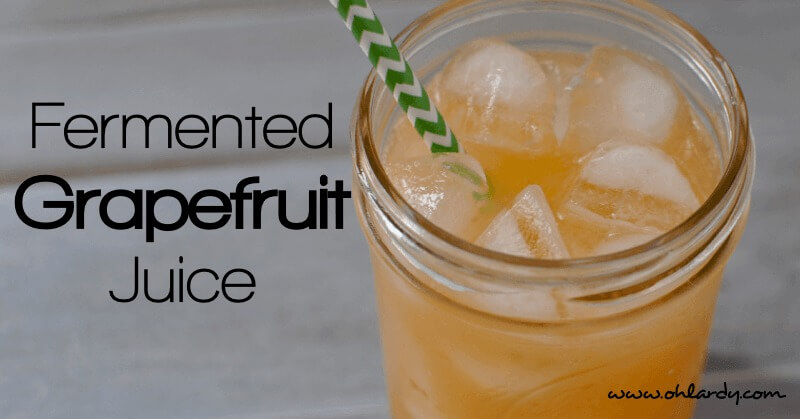This detailed photograph showcases a mason jar filled with orange-yellow fermented grapefruit juice, generously packed with ice cubes. Emerging from the jar is a striking green and white striped straw. To the left, bold black text reads "fermented grapefruit juice," with "grapefruit" emphasized in thicker lettering. A cursive web address, www.ohlardy.com, graces the bottom right corner of the image. The background is an indistinct gray, possibly a table or tablecloth, blurred to keep the focus on the jar and the inviting beverage within.